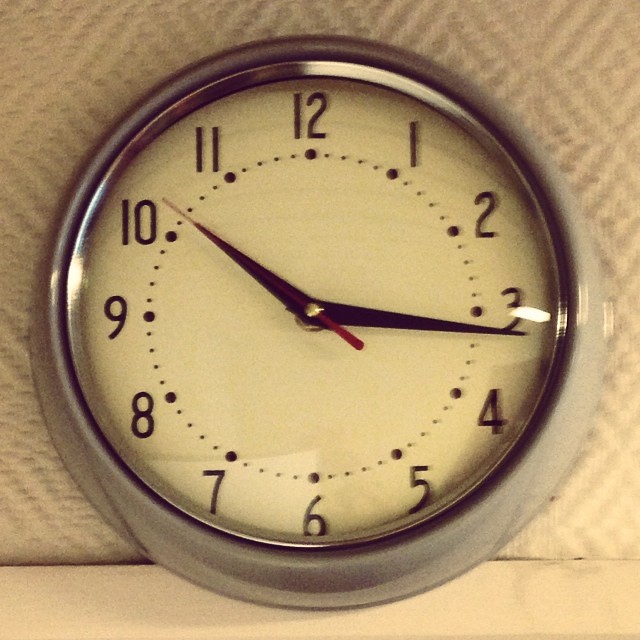A silver-framed wall clock, reminiscent of a polished dog bowl, is presently leaning against a roll of paper towels on a beige Formica counter, instead of hanging on a wall. The clock features a somewhat aged, off-white face with black numerals clearly marking 12 through 11. It has a black hour hand, a black minute hand, and a distinctive red second hand, currently indicating the time as 10:16. The overall composition highlights the juxtaposition of the sleek metallic clock against the casual, everyday kitchen setting.